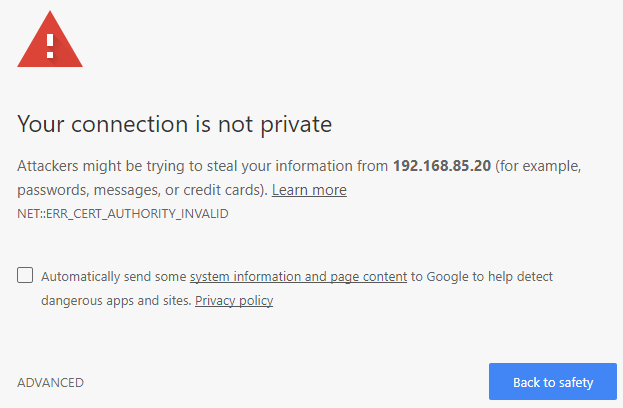This is a detailed screenshot of a security alert from Google Chrome. The alert is displayed in a gray box. At the top left corner of the box, there is a red triangle icon with a white exclamation point inside. Directly below this icon, in large gray text, are the words "Your connection is not private." The message warns that "Attackers might be trying to steal your information from 192.168.85.20," followed by examples such as passwords, messages, or credit card details.

Adjacent to this warning is a "Learn more" link. An error code is also present, which reads: "NET::ERR_CERT_AUTHORITY_INVALID." Below the error code is a checkbox option that reads, "Automatically send some system information and page content to Google to help detect dangerous apps and sites," along with a link to the Privacy Policy.

At the bottom right of the gray box is a blue button labeled "Back to safety," which users can click to return to a safer web environment.